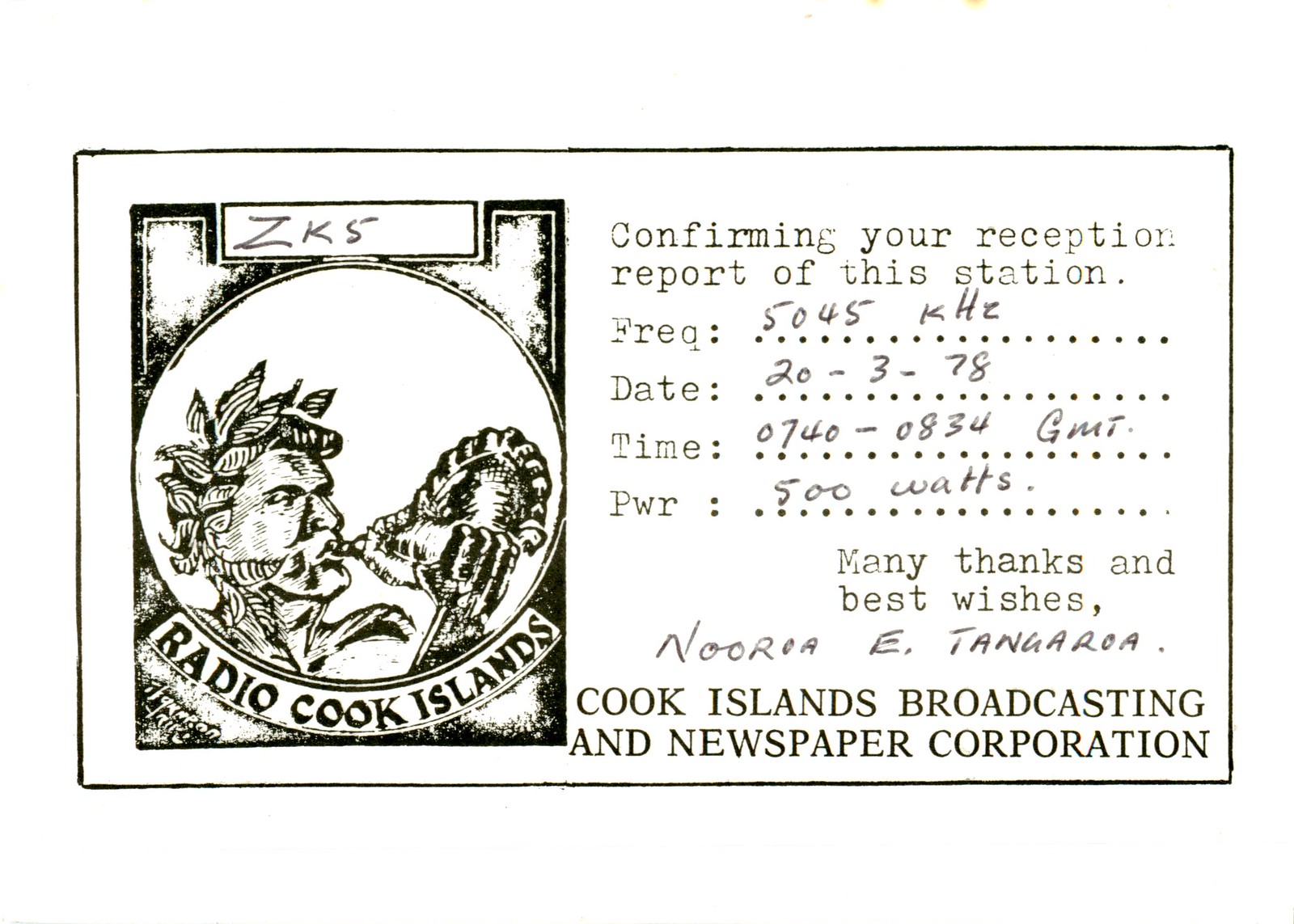This image depicts a digital card or verification slip featuring information related to a radio reception report. The background is primarily white, with elements in light pink or brown. On the left side, the card prominently displays "ZK5" at the top, followed by "Radio Cook Islands". Below this, an illustrated design shows a man appearing to blow into a conch shell, with artistic elements resembling wheat. The design might also symbolize "radio-focused eye movement".

On the right side, the card contains textual details under the heading, "Cook Islands Broadcasting and Newspaper Corporation." It formally acknowledges the reception report of the station, detailing the specifics as follows:
- FREQ: 5045KHZ, handwritten
- Date: 20-3-78, handwritten
- Time: 0740-0834GMT, handwritten
- PWR: 500 watts, handwritten

The card concludes with a message of gratitude and best wishes, signed by "Nora E. Tangaroa". The entire card is presented in black and white, giving it a classic, formal appearance.